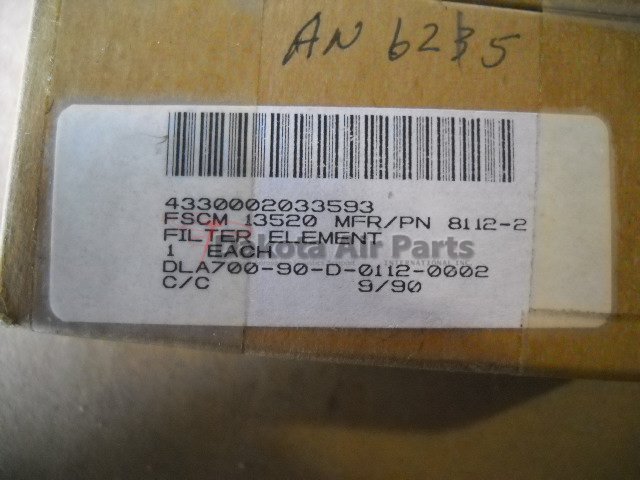The image showcases a brown box featuring a barcode label. Near the top of the box, the text "AN B235" is visible, although there is a faint vertical line through the "3" and what might be a "B" could also be a "6," making it somewhat ambiguous. The barcode on the label consists of vertical black and white stripes. Centered below the barcode is the company name, "Dakota Air Parts." The label contains numerous lines of text and numbers. The top line reads "4330002033593." Below this is "FSCM 13520 MFR/PN 8112-2." Further down, the text "Filter Element" is displayed, followed by another line with "DLA700-90-D-0112-0002." The final line contains "C/C," a large space, and "9/90."